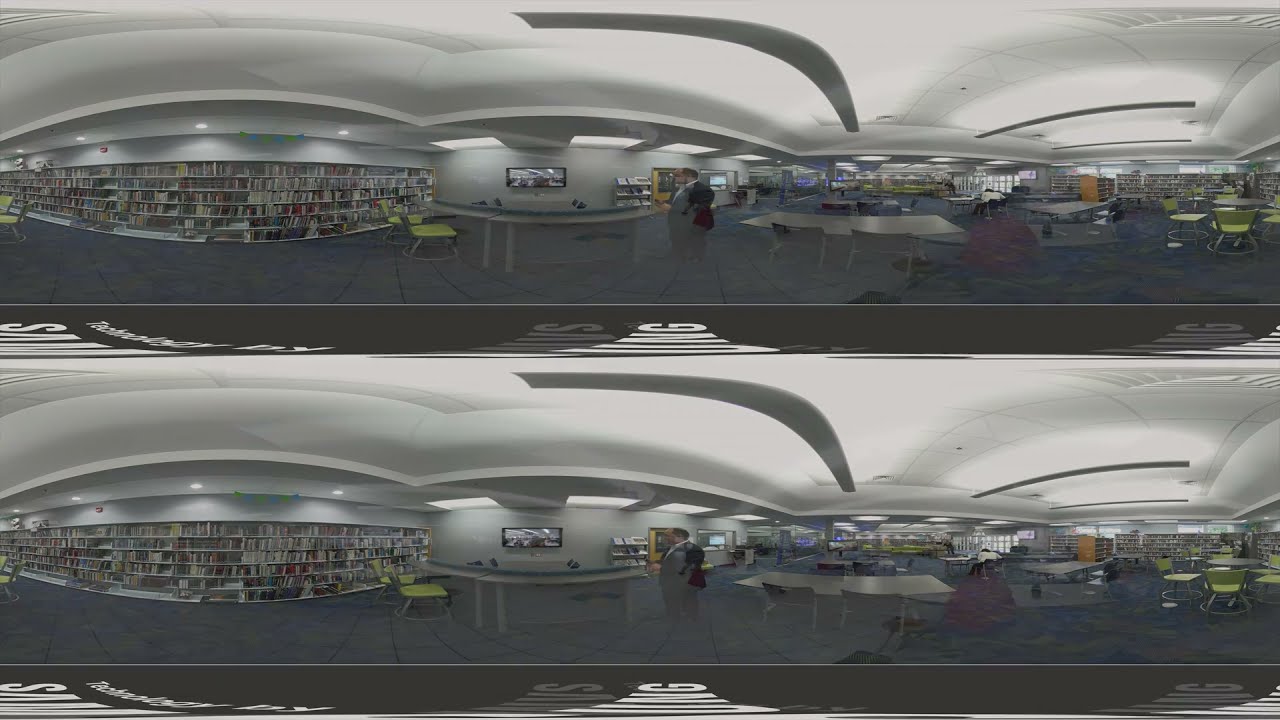The photograph, a horizontal and nearly square image, captures the interior of a school library with a focus on a central male figure. The man, who is bald and dressed in a blue suit with a white shirt and brown leather shoes, is addressing the camera with a gesturing hand that holds an object. The library's flooring features dark blue carpeting with a yellow-grey pattern. 

Around the room, several grey tables with blue and yellow chairs are visible, along with bookshelves lining the walls filled with books. A distinctive feature is a bar-like table area with yellow bar stools and a computer monitor. The well-lit space includes soft ceiling lights and mounted TV screens. In the background, there are a couple of people; one of them is a woman in a white shirt working on her computer at a table, seated by herself. The overall scene is bustling with the essence of a typical library setting.